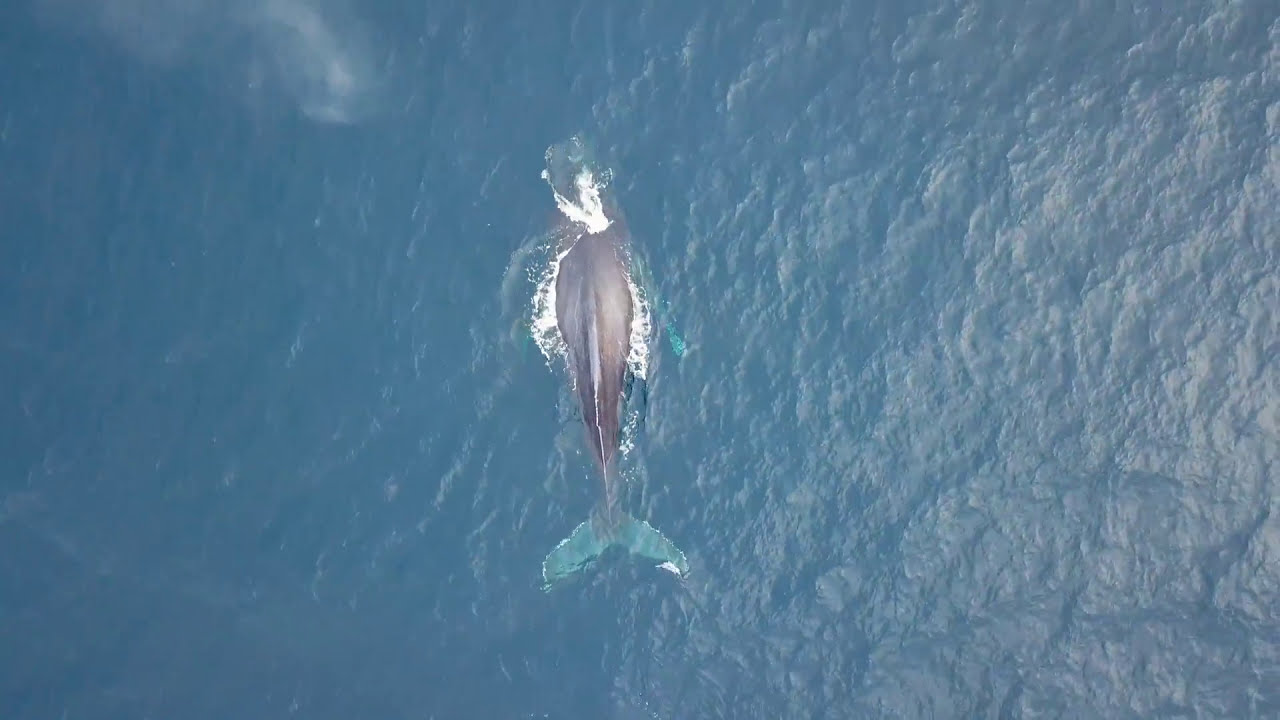A grayish-silver sea mammal, likely a whale, is captured in this aerial drone shot as it dives into a vast, open body of water. The whale's tail is still in the water, while its arched back and spine are visible above the surface. The water is calm and steel blue, disturbed only by the white splashes from the whale's movement. Sunlight brightens the scene, indicating it is a sunny day. There are no other animals or objects around, emphasizing the solitude of this majestic creature in its natural habitat.